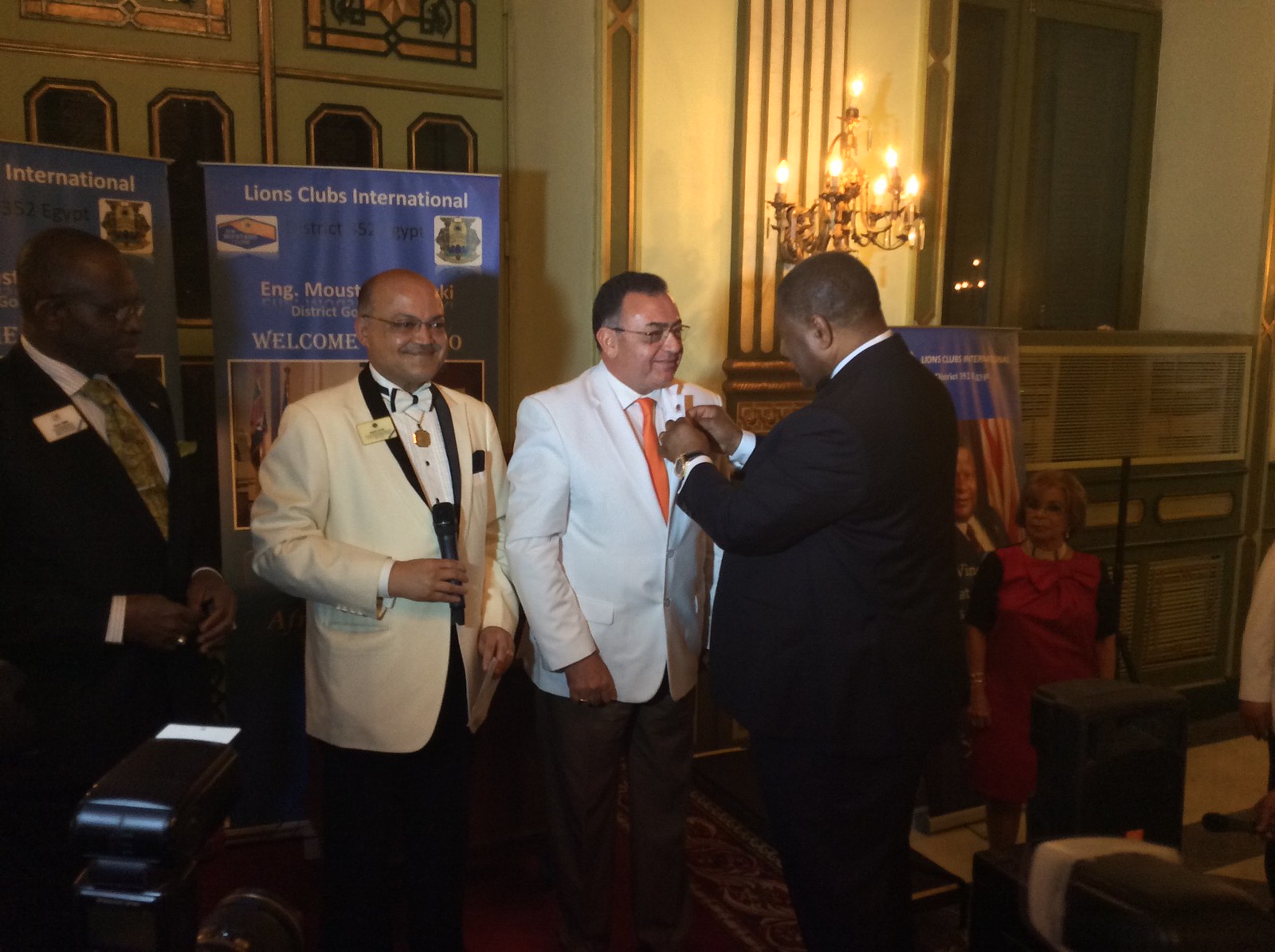In this color photograph, a ceremonial event for the Lions Club International is taking place in an ornate, elegant room with beige and gold walls and a chandelier. Four men are the focal point of the image, positioned on a pedestal or stage. From left to right, the first man is wearing a dark suit with a light-colored tie, his gaze directed at the pinning ceremony. Next to him, a bespectacled man in a white suit jacket with a black lapel and white bowtie holds a microphone. The central figure, a Latino man in a white jacket, black pants, and bright orange tie, is smiling as a black man in a dark suit pins a button or badge to his lapel. In the background, a woman in a red coat and another man in a dark suit with a brown tie look on. Two banners behind them read "Lions Club International Welcome You," and a large window highlights the room's luxurious decor and immaculate carpeting.